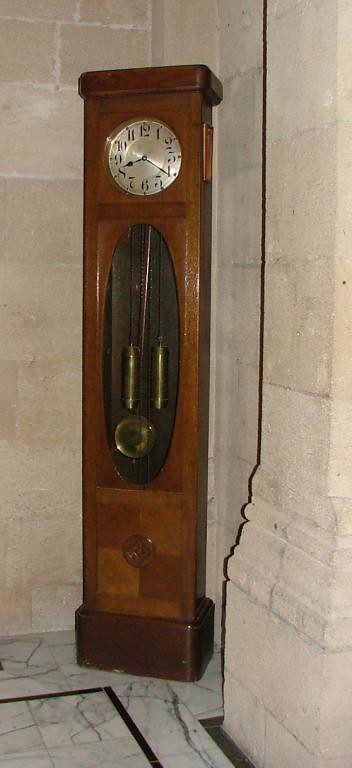This image depicts a brown grandfather clock showing the time as 8:20, though it's unclear if it's AM or PM due to the absence of windows. The clock is positioned on a marble floor with a distinct black border towards the center. The walls surrounding the clock are constructed from concrete blocks, suggesting the setting could be a castle or European mansion, rather than a typical modern home. The rectangular clock, devoid of ornate detailing, stands in stark contrast to the grandeur of the marble floor and sturdy, exposed joint walls.